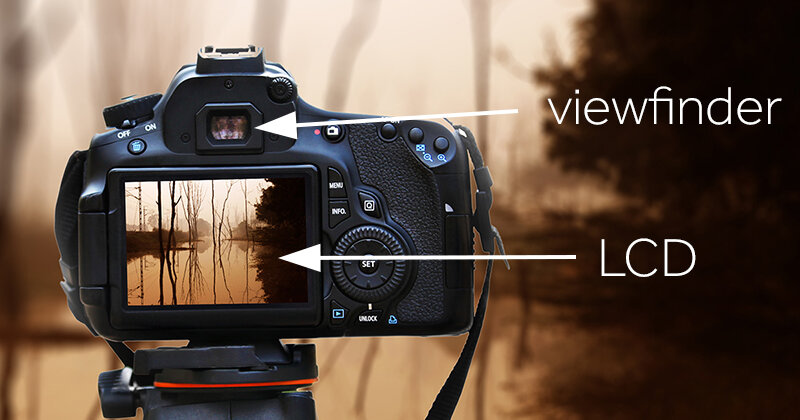The photograph shows a professional-grade digital camera mounted on a tripod, although the tripod's bottom is not visible. The camera, directed towards a swampy landscape with bare trees and a conifer to the right, is capturing this scene in its viewfinder and on its LCD screen. The image includes text labels with arrows pointing out the camera’s key components: the "viewfinder" and the "LCD" screen. The blurred wilderness background emphasizes the camera's capability, suggesting it might be used for an advertisement or demonstration of the camera's features.